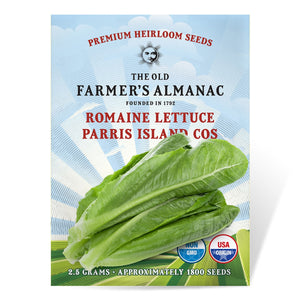This image depicts a vertically oriented package for premium heirloom seeds featuring a predominantly blue background. At the top, "Premium Heirloom Seeds" is boldly displayed in red letters. Below this, there is an illustration of the sun emitting rays, surrounded by the iconic black text, "The Old Farmer's Almanac, founded in 1792." Centered beneath is the product name, "Romaine Lettuce, Paris Island COS," written in striking red letters.

The central image showcases several lush, green leaves of romaine lettuce, with varying shades of green and intricate light green veins. Two logos appear near the bottom: one, encased in a red-bordered circle, affirms the seeds' USA origin; the other, contained within a blue circle, remains difficult to decipher. Finally, at the very bottom, the text indicates the package holds 2.5 grams of seeds, approximately 1,800 in total. The background subtly features a farm landscape, suggesting fields of growing lettuce.